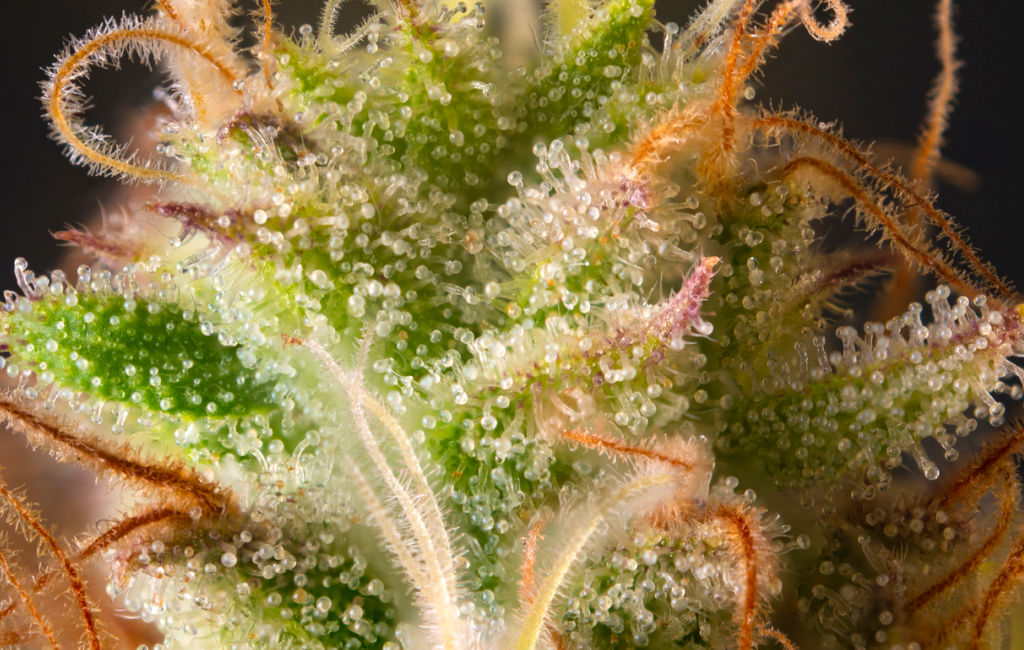This image captures a mysterious sea creature, detailed with a mix of vibrant and intricate features. Dominantly centered is a greenish, cactus-like main body adorned with transparent, bulbous structures. Surrounding this central form are numerous tentacles, exhibiting a diversity of colors and textures. Thick greenish tendrils extend outward, some horizontally to the left and right while others rise vertically, each tipped with white, ball-like protrusions. Interspersed are string-like orange tentacles, densely populated with tiny, hair-like follicles that give them a fuzzy appearance. These orange tendrils twist and curl in various directions, some looping over themselves, creating a dynamic visual effect. Additionally, a few thin white and brown tendrils, some with a bottle-brush appearance, emanate from the bottom, curling at the tops and sides. The backdrop is a deep midnight blue, providing a stark contrast that enhances the vividness of the creature, though it darkens towards the upper left and right corners, further emphasizing the central focus on this unique and intricate sea life. The entire scene is set against this dark, aquatic background, suggesting an underwater environment and adding a sense of depth and mystery to the image.